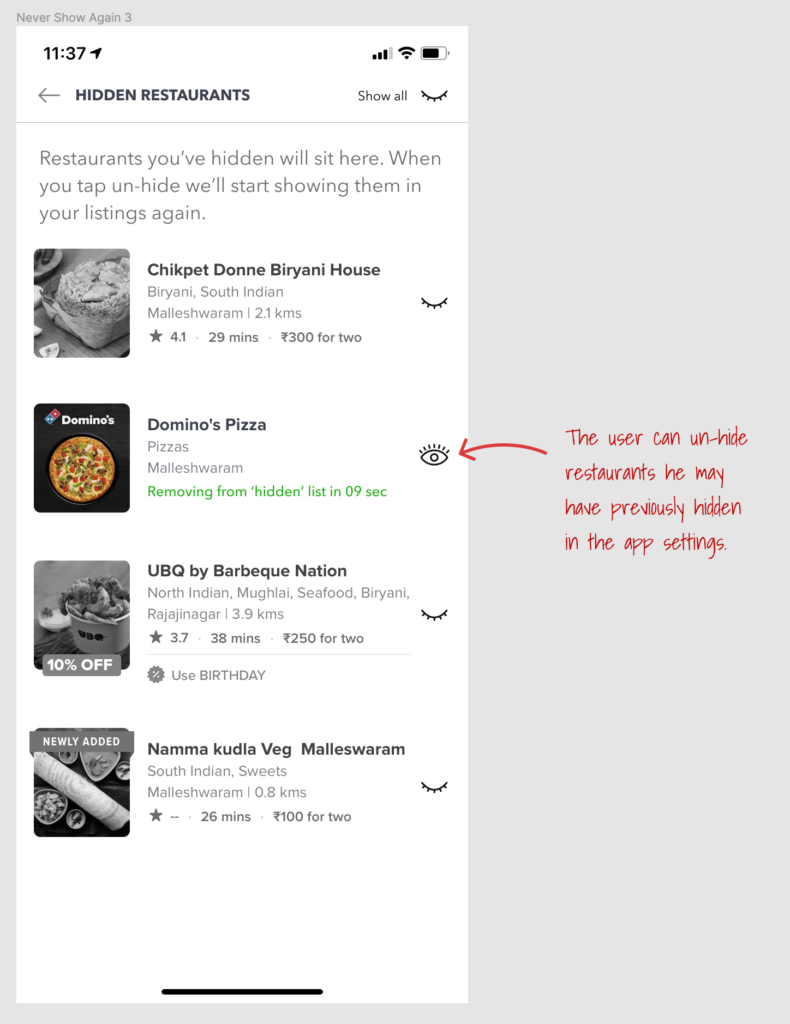This image is a detailed screenshot of a smartphone mounted on an off-white background page, showcasing a user-interface guide for unhiding restaurants in a specific app. 

The phone displays a screen with a white background, situated on the right half of the larger off-white background. Centered on the right-hand side of the image, there is red text in a handwritten style that reads, "The user can unhide restaurants he may have previously hidden in the app settings." Accompanying this text is a red arrow pointing left towards an icon of a wide-open eye.

At the top of the phone screen, the time reads 11:37, with indicators showing three strong Wi-Fi bars and three-quarters of the battery remaining. Below this, the title "Hidden Restaurants" appears in bold. Directly underneath, in lighter gray text, it states, "Restaurants you've hidden will sit here. When you tap Unhide, we'll start showing them in your listings again."

The listed restaurants are as follows, starting from top to bottom:
1. **Chick Pet Don Biryani House**, which is currently hidden.
2. **Domino's Pizza**, prominently displayed as unhidden and actively highlighted by the red arrow.
3. **UBQ by BBQ Nation**, listed but not highlighted.
4. **Nama Kula Veg Mao Swaram South Indian Sweets**, also listed but without any additional emphasis.

Overall, the image meticulously instructs users on how to manage the visibility of restaurant listings within the app, using visual cues and clear textual explanations.